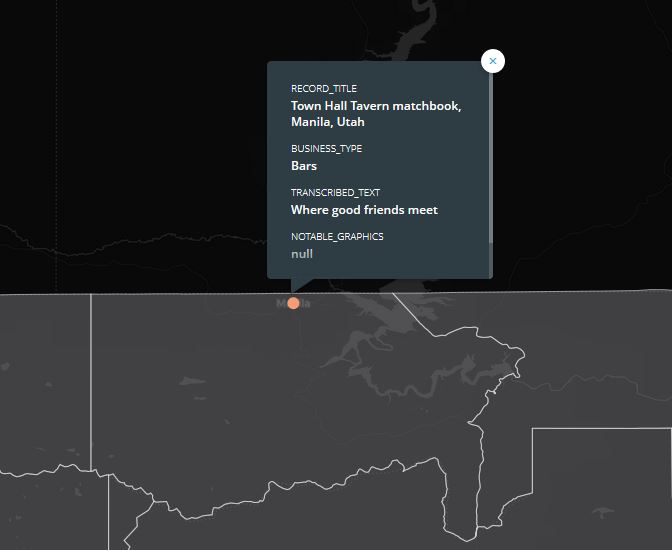In the video, the screen is divided into two sections, each displaying a different visual representation of a map. The top half of the map is rendered in dark black with some distinct lines that likely indicate rivers or other geographical features. There is a highlighted annotation bubble above this dark section, which contains the following text:

- "record title: record_title_town_hall_tavern_matchbook, Manila, Utah"
- "business_type: bars"
- "transcribe_text: Where good friends meet."
- "notable_graphics: button null"

Meanwhile, the bottom half of the map is presented in a lighter gray color. This section appears to be a more detailed version of the same map, featuring white lines that delineate different areas. These lines may represent state or regional boundaries. There are also visible indicators of bodies of water within this gray section.

A notable feature is a small orange dot which appears to mark the location of Manila on the map. From this dot, a line extends to the annotation bubble that provides further information about the location and its significance. The bubble clearly states "Manila," suggesting that this part of the map is focused on detailing an area in Utah.